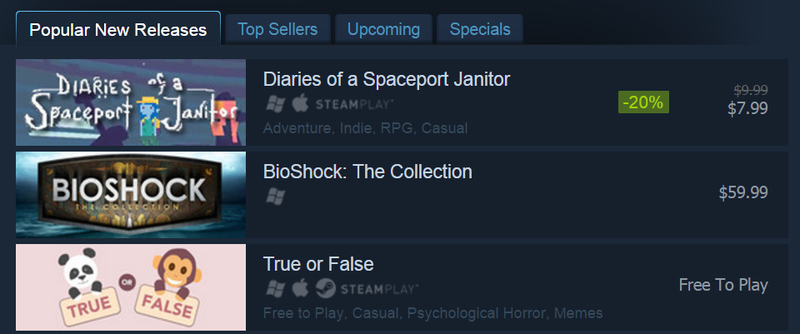The webpage features a navy background with several toggle options at the top. The currently selected option, "Popular New Releases," is highlighted in white text, against a box background matching the page’s navy hue. Adjacent toggle labels include "Top Sellers" in blue font, followed by "Upcoming" and "Specials."

In the "Popular New Releases" section, three images correspond to individual titles:

1. "Diaries of a Spaceport Janitor" showcases a quirky font with a blue caricature beside a red caricature. This title is currently 20% off, marked in a green box, with the discounted price of $7.99.
2. "Bioshock" presents its title in bold white letters on a brown-stamped background, referring specifically to "Bioshock: The Collection," priced at $59.99.
3. "True or False" features a pink image with cartoon characters—a panda bear holding the word "True" and a monkey holding "False." This game is listed as free to play.

Each title is paired with its respective image and pricing information, offering a clear snapshot of the latest releases.